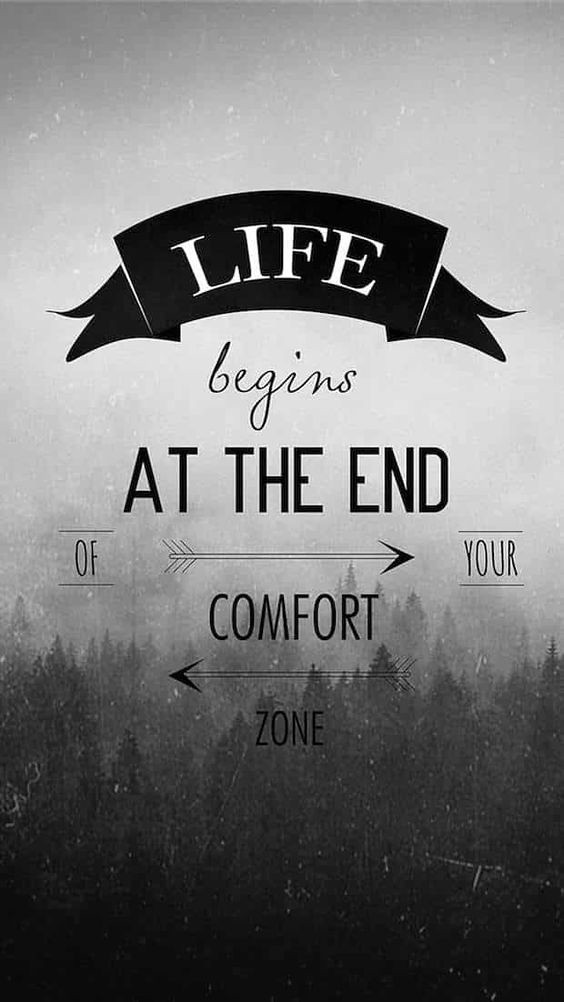This image appears to be a vertical cover, possibly for a movie or book, featuring an inspirational quote. The background of the image is primarily black and white and depicts a dense forest, likely pine trees, viewed from a high vantage point on a mountain. The photograph at the bottom of the image showcases these trees reaching upward into a foggy atmosphere, with the fog becoming denser as it ascends into the sky. 

At the top of the image, there is a black ribbon with white text that reads "Life." Below this ribbon, the word "begins" is written in cursive. Further down, the phrase "the end" is marked in bold black text. Positioned horizontally around an arrow pointing to the right are the words "of" on the left and "your" on the right. Beneath this is another black arrow, this time pointing to the left, directing the eye towards the concluding part of the quote: "comfort zone." Together, the text on the image reads: "Life begins at the end of your comfort zone," accentuated by directional arrows.